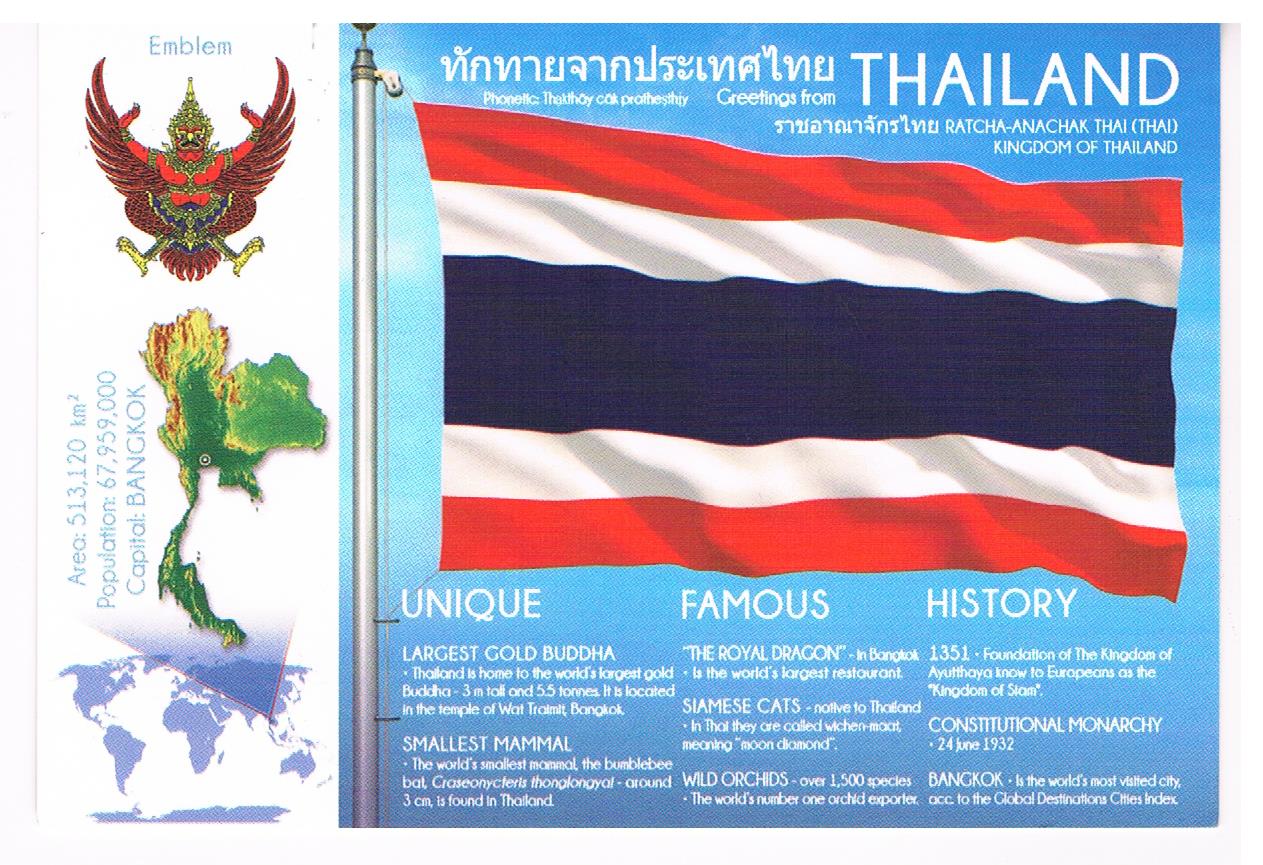This informational graphic about Thailand features detailed elements across the entire card. Dominating the right-hand side is the national flag, characterized by a large, horizontal navy blue stripe centered between two white stripes, each edged by red stripes. Just below the flag, "Thailand" is prominently labeled, accompanied by characters in the Thai language. The emblem of Thailand, a mythical bird with a crown representing the country's royal heritage, is also positioned at the top right.

The graphic is divided into sections showcasing various aspects of Thai culture and history. The "unique" section highlights wonders such as the largest gold Buddha and the smallest mammal. Centrally, the "famous" section lists the royal dragon, Siamese cats, and wild orchids. The "history" segment mentions key historical dates: the foundation of the Kingdom of Ayutthaya in 1351 and the establishment of the constitutional monarchy on June 24, 1932. Additionally, Bangkok is noted as the world's most visited city according to the Global Destinations Cities Index.

On the left side, a detailed map of Thailand shows the country's area of 513,120 square kilometers, a population of 67,959,000, and designates Bangkok as the capital. Adjacent to this map is a smaller global map in light blue, giving a geographical context.